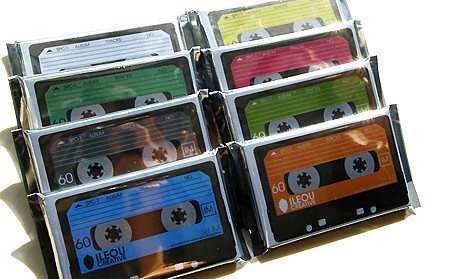The image features a neatly arranged display of eight cassette tapes, set against a white background. The cassettes are organized in two rows of four, creating a grid-like formation. Each cassette tape is encased in a transparent plastic container with a silver border, and they are casting noticeable shadows due to a light source positioned behind the camera. 

From left to right on the top row, the cassettes have colored labels as follows: white, yellow, green, and red. The bottom row continues with gray, green, blue, and orange cassettes. Upon closer inspection, the tapes bear the brand name "Illo Creative," with the label denoting "6-0" on the left and an "M" in a square box on the right side. Additional text such as "S-G-I" and what appears to be "N-O" is faintly visible on the tapes.

The vibrant colors and the orderly arrangement give the scene an artistic appearance, reminiscent of retro aesthetics, accentuated by the shadows cast on the pristine white background.